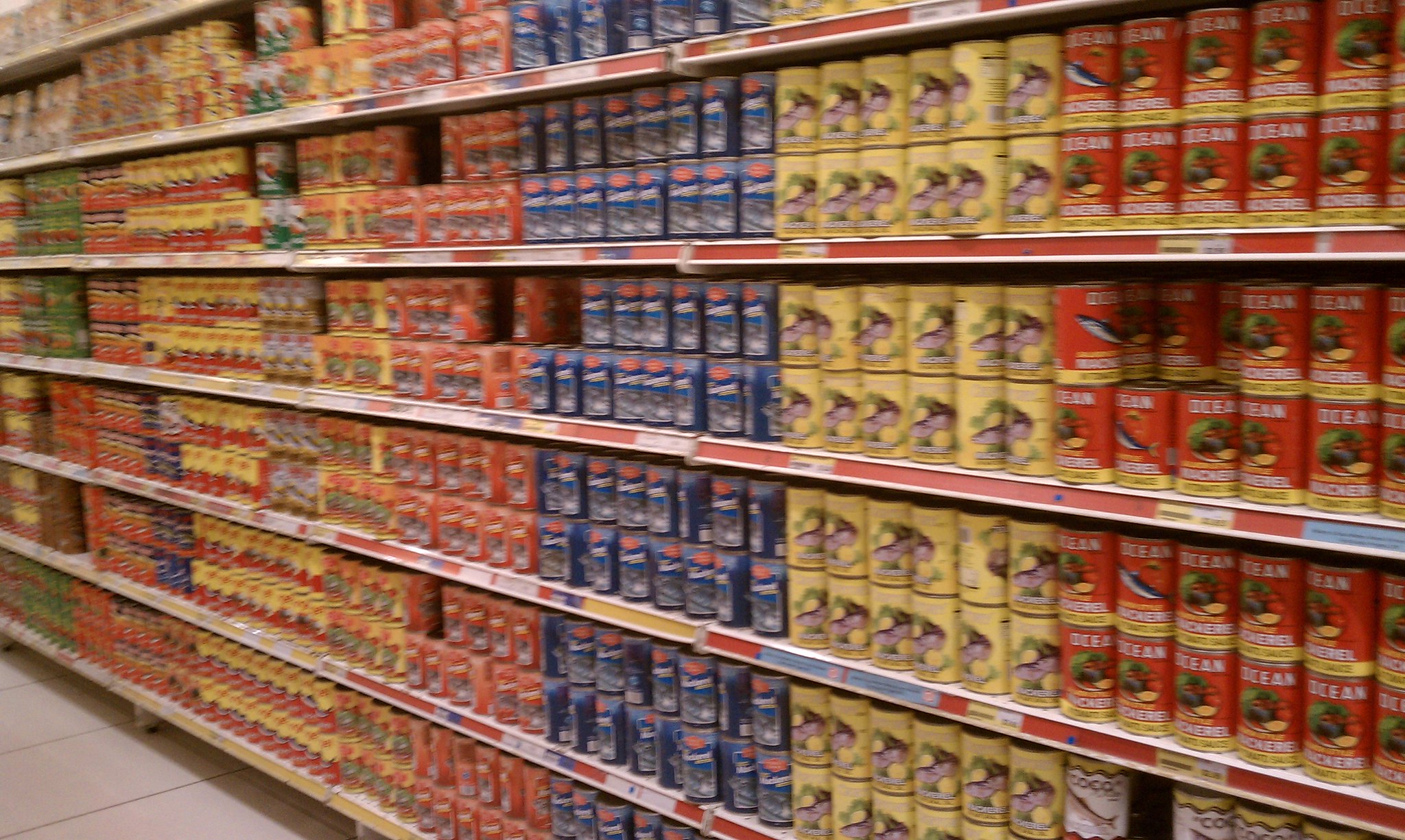The image depicts a supermarket aisle lined with an extensive array of canned goods. The aisle features large metal shelves with red fronts and yellow labels that display black lettering, which extend from the floor to the top shelf in columns. In the foreground, rows of red cans with yellow labels featuring the word "ocean" and an illustration of a fish are prominently visible, indicating they are likely canned fish. Adjacent to these are stacks of cans in blue, orange, yellow, and green, each grouping containing multiple copies of the same product. The photograph captures the shelves stretching off into the distance on the left side, emphasizing the vastness and variety of the stocked items. Despite the blur, the organizational pattern of the cans is clear, with colors shifting from red and yellow to blue, red, and back again, creating a vibrant mosaic of canned goods set against a tiled grocery store floor.